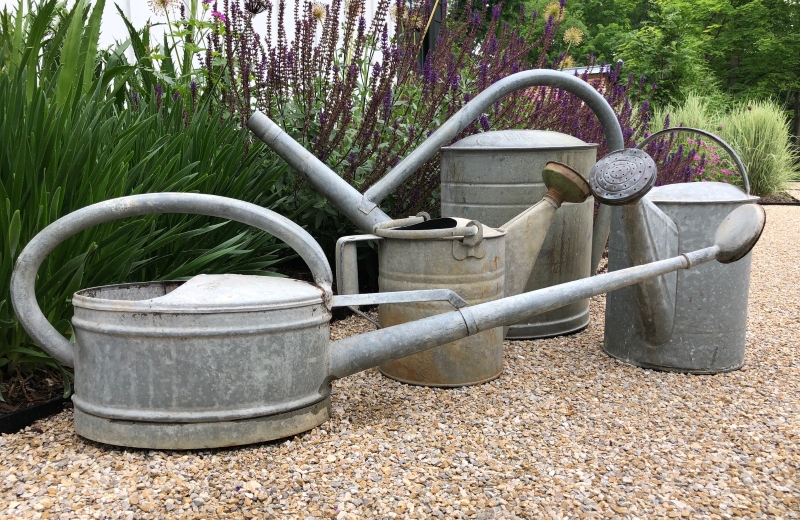The image is a color photograph taken during the daytime, capturing a rustic scene of four vintage metal watering cans, possibly from the 1940s or 50s, arranged on a light brown, white, and gray gravel ground. In the foreground, the can on the bottom left features a flat shape with a large handle arching from front to back, and it has a notably long spout. The other three cans have a traditional design with cylindrical bodies and varying heights, each equipped with circular shower head spouts, although one is missing its shower head. Behind the cans is a small garden adorned with a mix of plants, including green bushes and lilac-like flowers with striking dark purple blooms. The backdrop includes a white structure, likely a house, and a collection of taller green trees, some bearing yellow flowers, creating a serene and nostalgic garden scene.